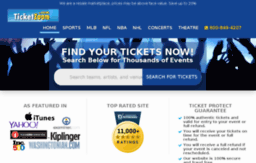This image is a screenshot of a concert website with a predominantly dark blue upper navigation bar that stretches horizontally across the top of the page. At the top center of this bar, there's white text displaying the website name or logo. On the left-hand side of this bar, there is a button resembling a small banner that reads "TicketZoom"—with "Ticket" in white font and "Zoom" in yellow font, presented as one continuous word, with "Ticket" uniquely capitalized with a 'C'. 

In the middle section of the navigation bar, there is a menu with various categories listed in white font. These categories include "Home," "Concerts," "Sports," followed by specific subcategories like "MLB," "NFL," "NBA," "NHL," "Concerts," and "Theater." On the far right side of the bar, there is a phone number displayed in yellow font, providing a contact option for visitors. The overall compact design and small text size make it somewhat difficult to read when the image is blown up.